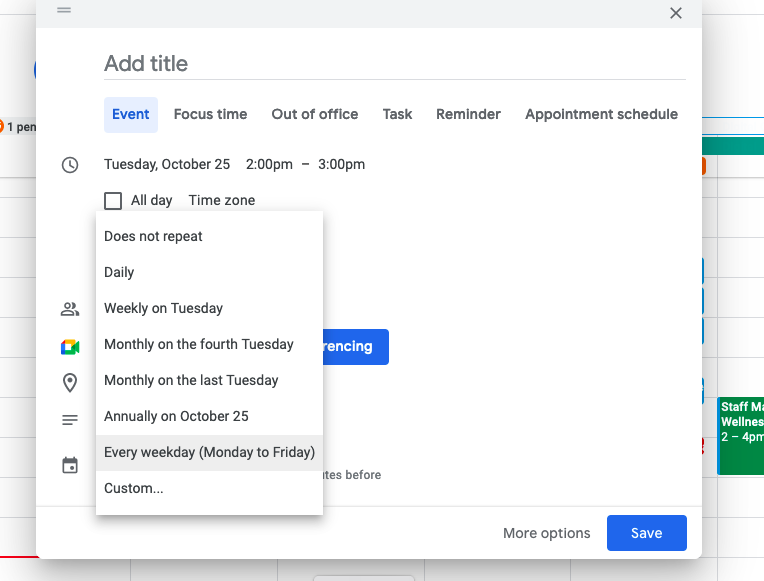Here is a cleaned-up and detailed descriptive caption for the image:

---

This image features a screenshot of a website with a pop-up tab overlaying the content. On the left side of the screen, there is a glimpse of the website, which has a white background. About two inches from the top, there are some text lines visible. There's a gray side tab labeled in black with the letters "P-E-N."

On the right side of the screenshot, there is a partially visible green rectangle about an inch from the bottom, displaying white text that reads "staff M." Below that, the word "wellness" is visible, though it's missing its final "S," followed by "2 to 4 P-M."

The pop-up tab itself has a light gray top border. At the top-left, there are two horizontal black lines, and at the top-right, there's a black "X." Directly below, about an inch from the left edge, bold black text reads "Add Title." Blue text below this reads "Event," encased in a light blue rectangle. Next, black lettering spans to the right of the pop-up, listing "Focus Time,” “Out of Task,” “Task,” “Reminder,” and “Appointment Schedule."

Below these options, the text says "Tuesday, October 25th, 2 P-M-3 P-M," accompanied by a small time icon to the left. Beneath this section, there is a square gray-bordered area with white text that reads "All Day" and next to it, "Time Zone."

Another pop-up tab appears within the main pop-up, featuring scheduling options. This tab is white with black text that lists various repeating events: "Does not repeat,” “Daily,” “Weekly on Tuesday,” “Monthly on the fourth Tuesday,” “Monthly on the last Tuesday,” “Annually on the 25th.” It is outlined with a gray rectangle, containing options like "Every weekday, Monday to Friday," and "Six Customs, where it says Weekly on Tuesday." Five vertical icons are positioned to the left of these texts.

In the middle of the pop-up tab, a partial blue rectangle shows the letters "E-N-C-I-N-G" in white. At the bottom right corner, a blue button says "Save" in white, and to its left, a black text button reads "More options."

---

This detailed caption captures the various elements presented in the screenshot, structuring the information for clarity and ease of understanding.